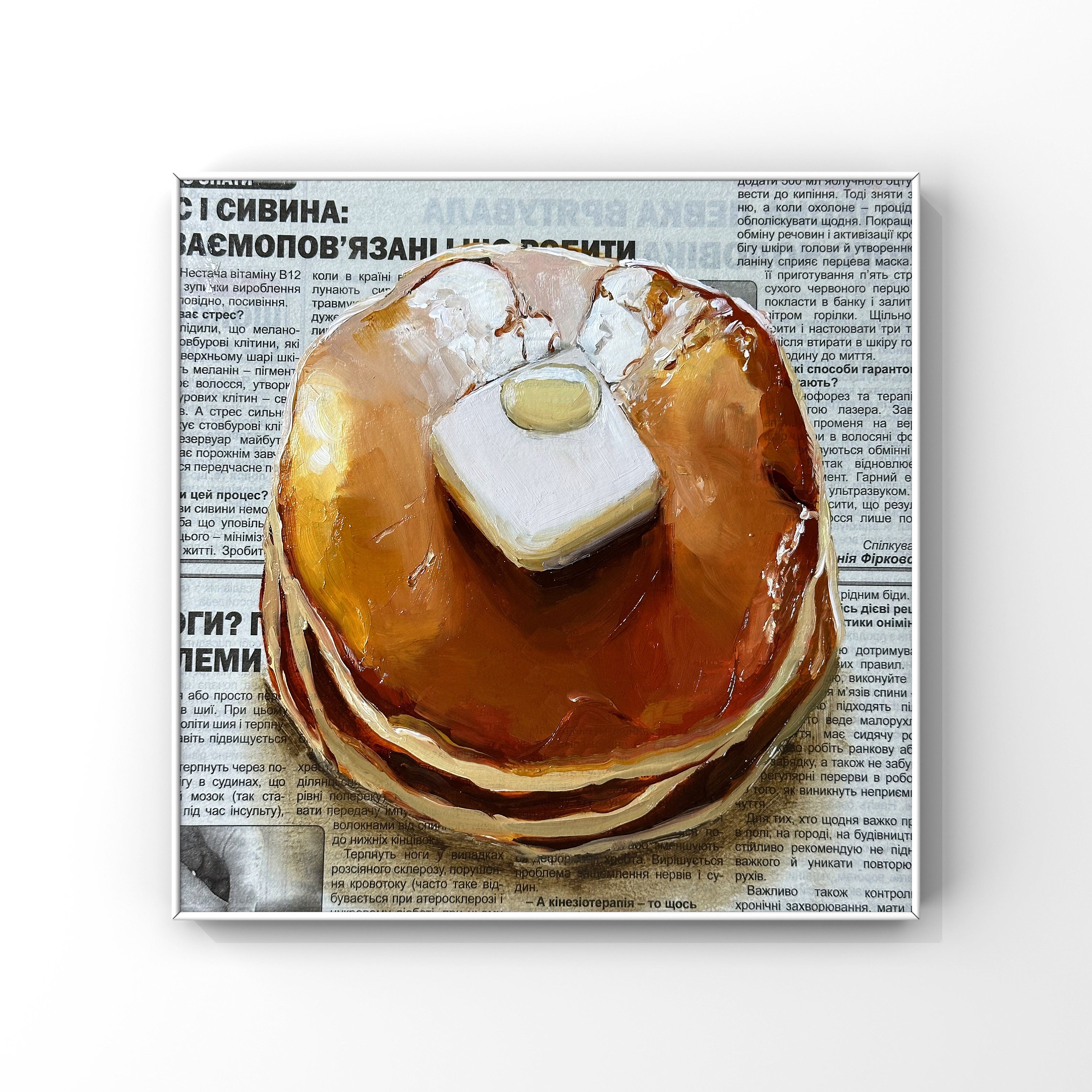The image depicts a still life scene featuring a stack of three or four pancakes, perfectly centered on a small, clear glass plate that is almost the same diameter as the pancakes themselves. The plate is situated on a square clipping of a Russian newspaper, adding an unusual yet intriguing backdrop. The focal point of the composition is the stack of golden-brown pancakes with a slightly darker edge, crowned with a large, partially melted square of butter. The butter appears to be slowly melting, mixing with a glossy layer of syrup—either maple or a clear variety—that cascades down the sides of the pancakes. This artistic portrayal blurs the line between painting and photography, offering a hyper-realistic yet stylized representation of a classic breakfast. The entire scene is framed minimally, providing a clear view of the newspaper's Cyrillic text under the transparent plate, thus suggesting a cultural or perhaps nostalgic context to the meal.